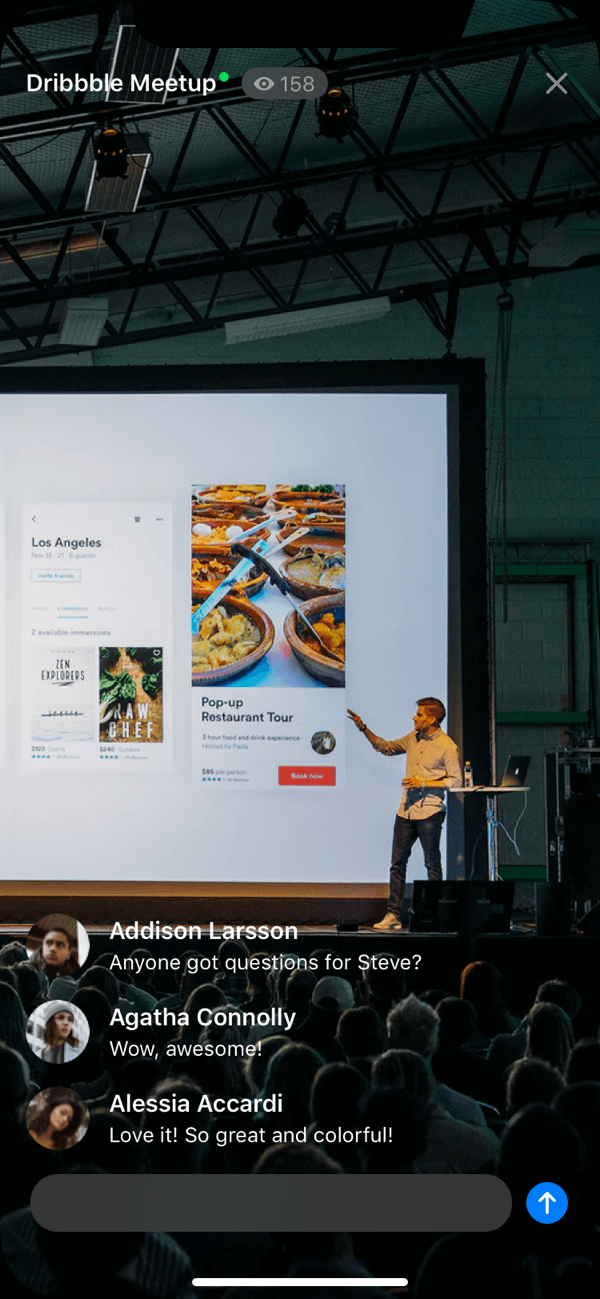The image shows a screen capture from a cell phone, highlighting a Dribble Meetup event. At the top of the screen, it displays "Dribble Meetup," along with a view count of 158. In the background, a person stands on stage, giving a speech. The speaker is dressed in a yellowish shirt, black pants, and matching yellowish shoes. Behind him, a large screen displays what appears to be cooking-related content, indicating he may be demonstrating or highlighting dishes. The screen prominently features the text "Pop-up Restaurant Tour" with the location noted as Los Angeles.

The audience is visible, attentively watching the screen behind the speaker, with some scaffolding visible above them. Below the main event scene, the screenshot captures three comments from attendees. Addison Larson's comment reads, "Anyone got questions for Steve?" followed by Agatha Conley stating, "Wow awesome," and Alyssa Akardi expressing, "Love it, so great and colorful." Profile pictures of the commenters can be seen to the left of their respective messages, adding a personal touch to the interactive chat.